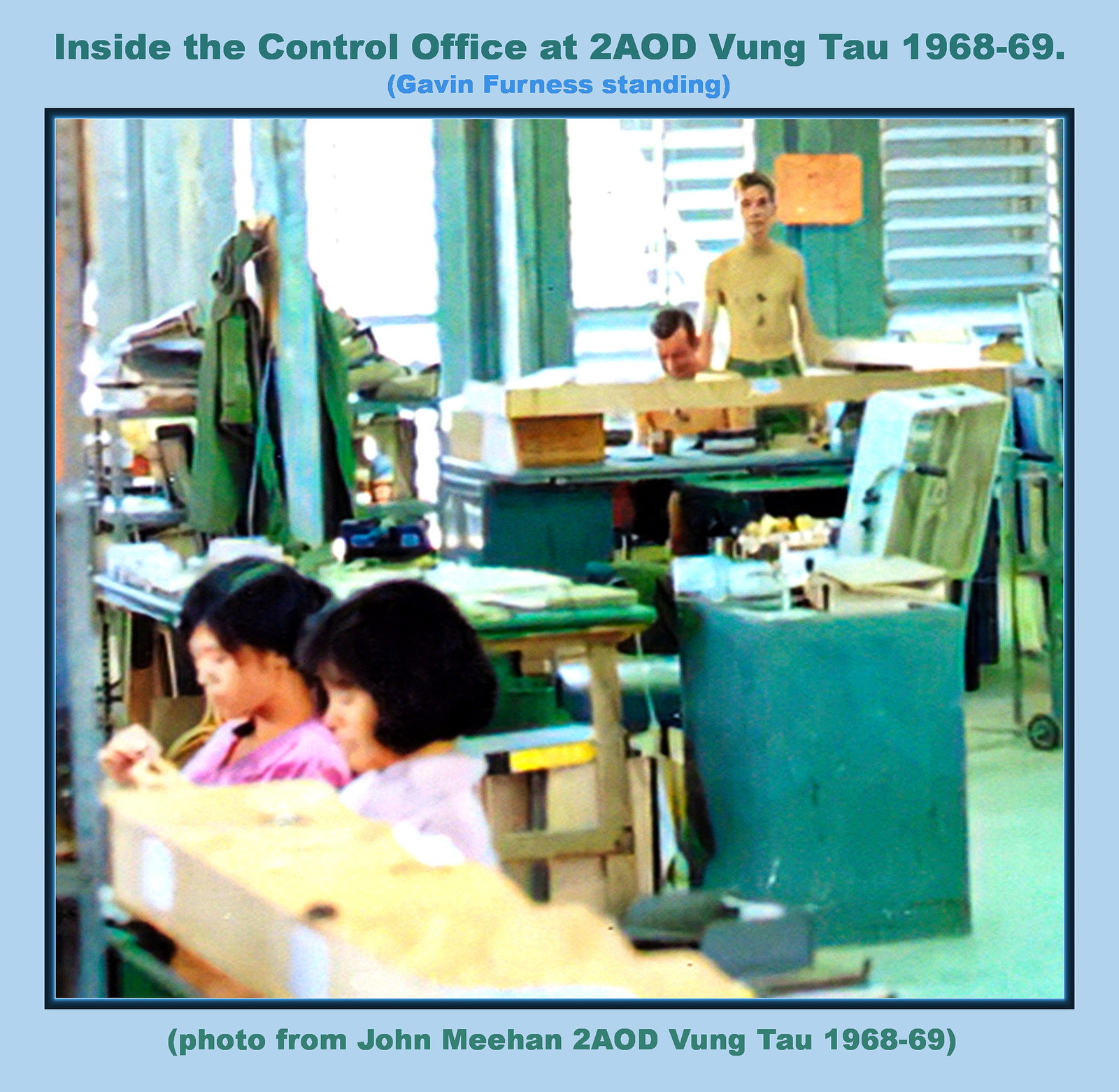The image depicts a vintage photograph from the Vietnam War era, specifically taken inside the control office at 2AOD, Vung Tau, between 1968 and 1969. The photograph is bordered by a black frame with captions indicating the details: "Inside the Control Office at 2AOD, Vung Tau, 1968-1969" at the top and noting "Gavin Furness standing" alongside the photo credit "Photo from John Meehan, 2AOD, Vung Tau, 1968-1969" at the bottom.

The setting appears to be an indoor, disheveled office or manufacturing environment with a prominent green color palette. The room is cluttered with various objects piled on shelves, tables, and benches, contributing to a sense of disarray. 

In the foreground, two young Asian women with dark hair are seated at a desk or table, looking down intently at their hands, suggesting they might be assembling or crafting something. Nearby, there is a cart holding several papers and miscellaneous items.

In the background, a shirtless man identified as Gavin Furness, who appears to be a soldier given his dog tags, stands in front of windows with blinds. Another shirtless man is seated at a desk. The overall ambiance of the photograph evokes a busy wartime office setting, reflecting the era and the activities within this control office during the Vietnam War.